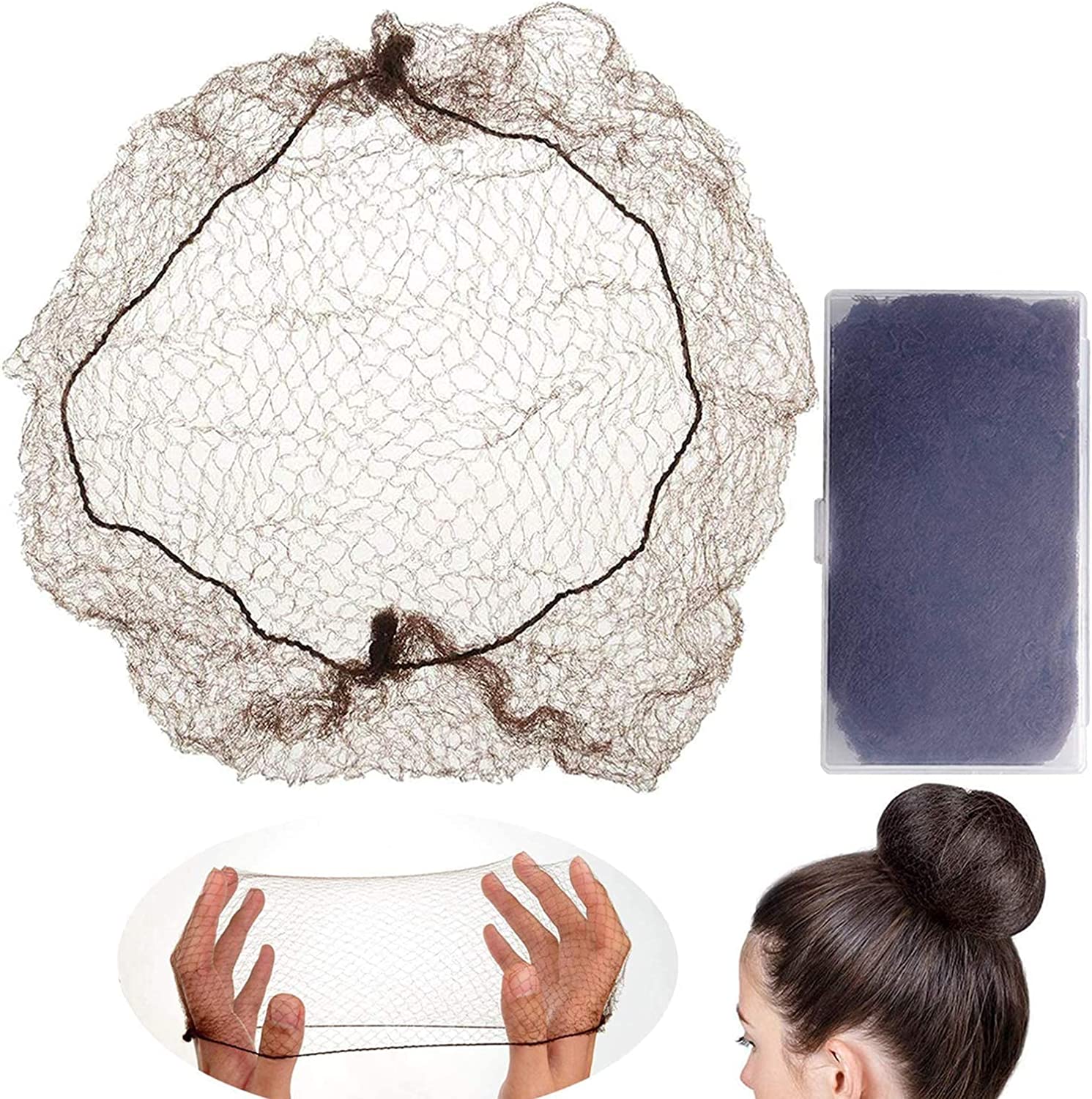The image is a comprehensive display of a black hairnet against a white background, presented in four distinct sections. The top left section features a fully opened hairnet, showcasing its intricate weave, circular shape, and the elastic band that secures it on the head. Adjacent to it, on the right, is a slightly purplish-gray, snap-closure case adorned with subtle filigree edging at the corners, resembling a small change purse, which is intended for storing the hairnet. The bottom left quadrant highlights two hands stretching the hairnet to emphasize its extensibility and weave pattern. Finally, the bottom right segment displays a side view of a female Caucasian with long brown hair neatly tied into a high bun, covered securely by the hairnet. The hairnet is shown to tightly conform to the shape of the bun, demonstrating its practical use.